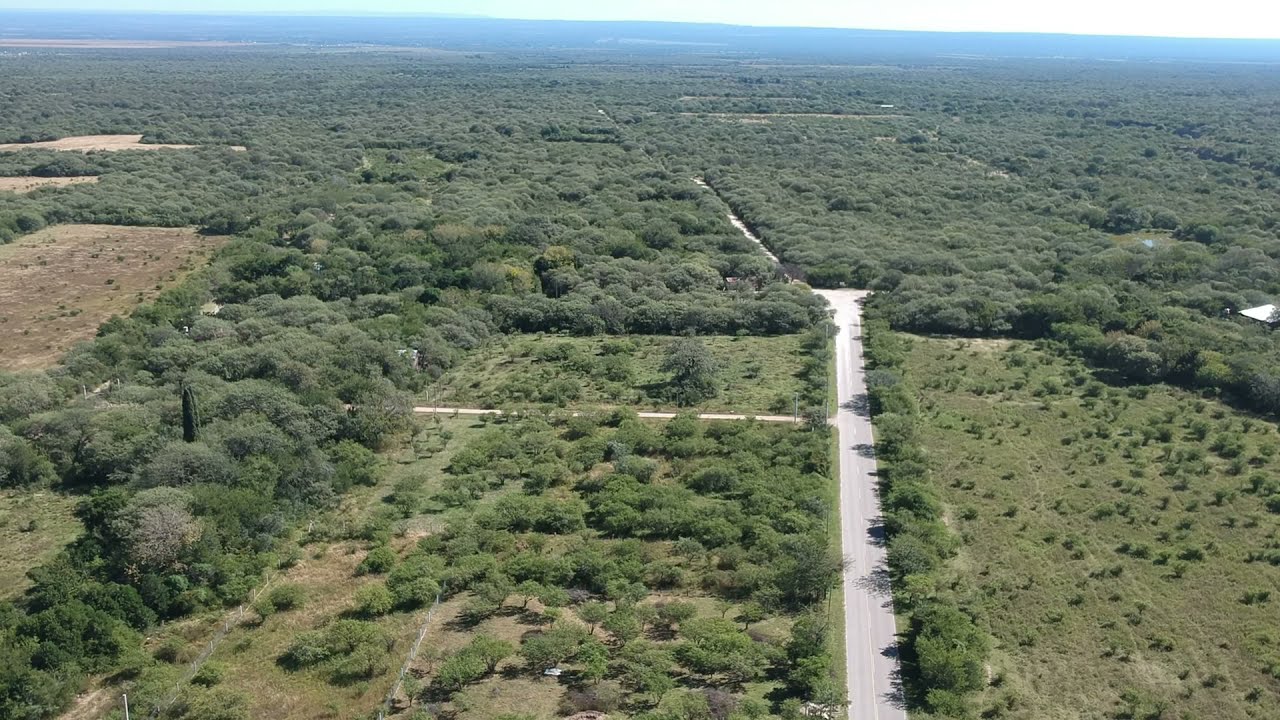This aerial drone photograph in landscape orientation captures a verdant rural area teeming with greenery. Dominating the scene is a straight gray road, slightly right of center, running from the bottom midsection and dog-legging to the left as it vanishes into the horizon. This road appears surrounded by dense clusters of vibrant green trees and overgrowth, interspersed with patches of open land and dirt fields. Another road intersects horizontally but doesn’t extend fully across the image. Alongside the primary road are lines of trees, giving the impression of a green corridor cutting through the thick forest areas. In the distance, a low mountain range or perhaps a distant water body emerges as a narrow blue band against a white daytime sky, suggesting a sunny day. The photograph shows a dynamic blend of greens, browns, and blues, with notable elements like a tent-like structure on the right, adding to the rural tranquility of the landscape.